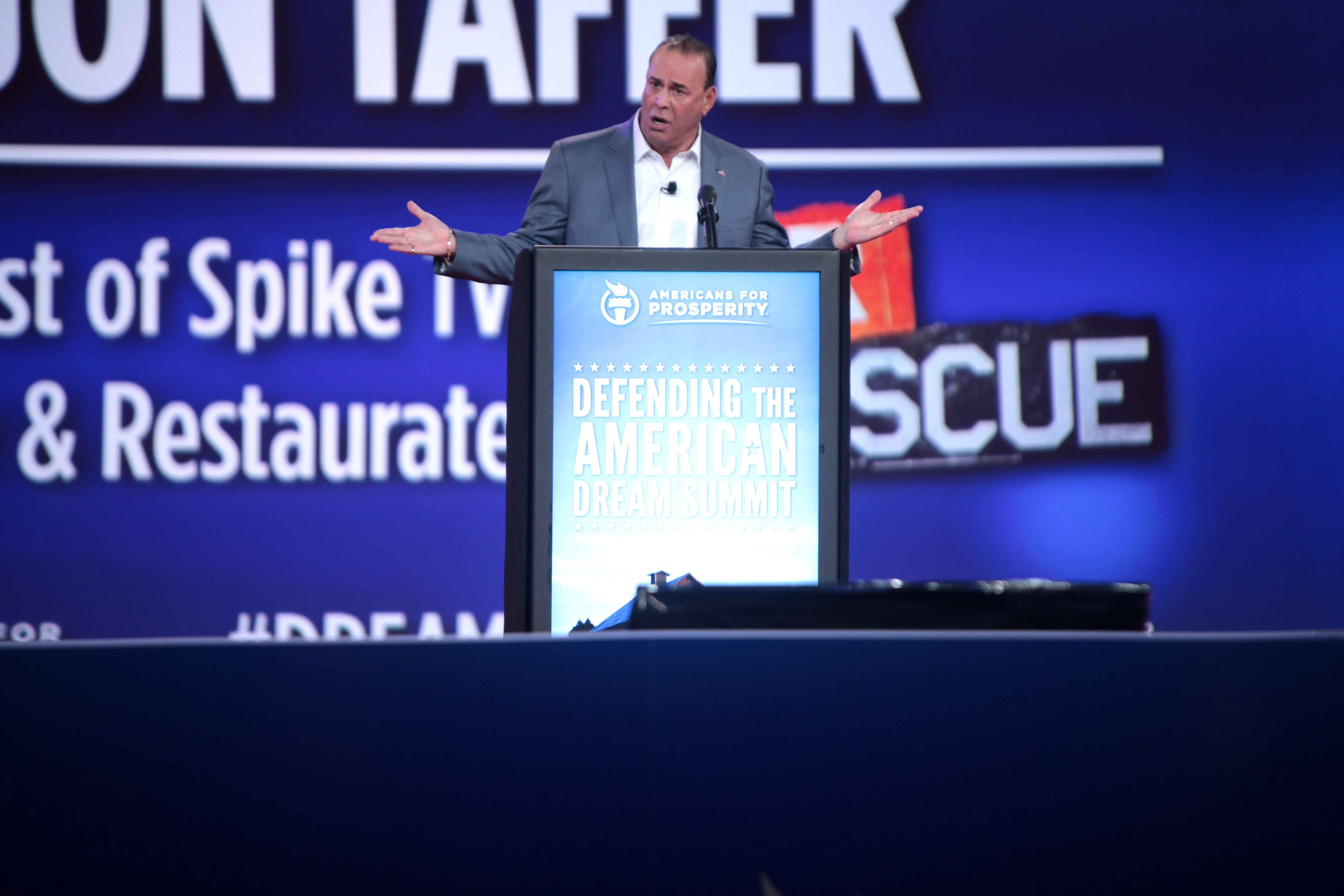This detailed photograph captures a man, likely a white male, standing on a stage at a podium, speaking passionately at an event. He is wearing a grayish-blue suit jacket over a white button-down shirt, with a black clip-on microphone affixed to it. The man, who is balding with short hair, has his arms bent at 90 degrees at the elbows, palms facing upwards, as though questioning or emphasizing a point to the crowd. He appears somewhat frustrated or intense in his expression. 

The podium in front of him prominently displays a blue sign with white text reading "Americans for Prosperity, Defending the American Dream Summit," and features a circular symbol with a torch. Behind him, there's a large blue digital screen displaying white, partially cut-off text including fragments like "UBSPIKETV," "R-E-S-T-A-U-A-R-T-E," and "S-C-U-E." The atmosphere suggests a formal and significant gathering, likely focused on national or economic issues.